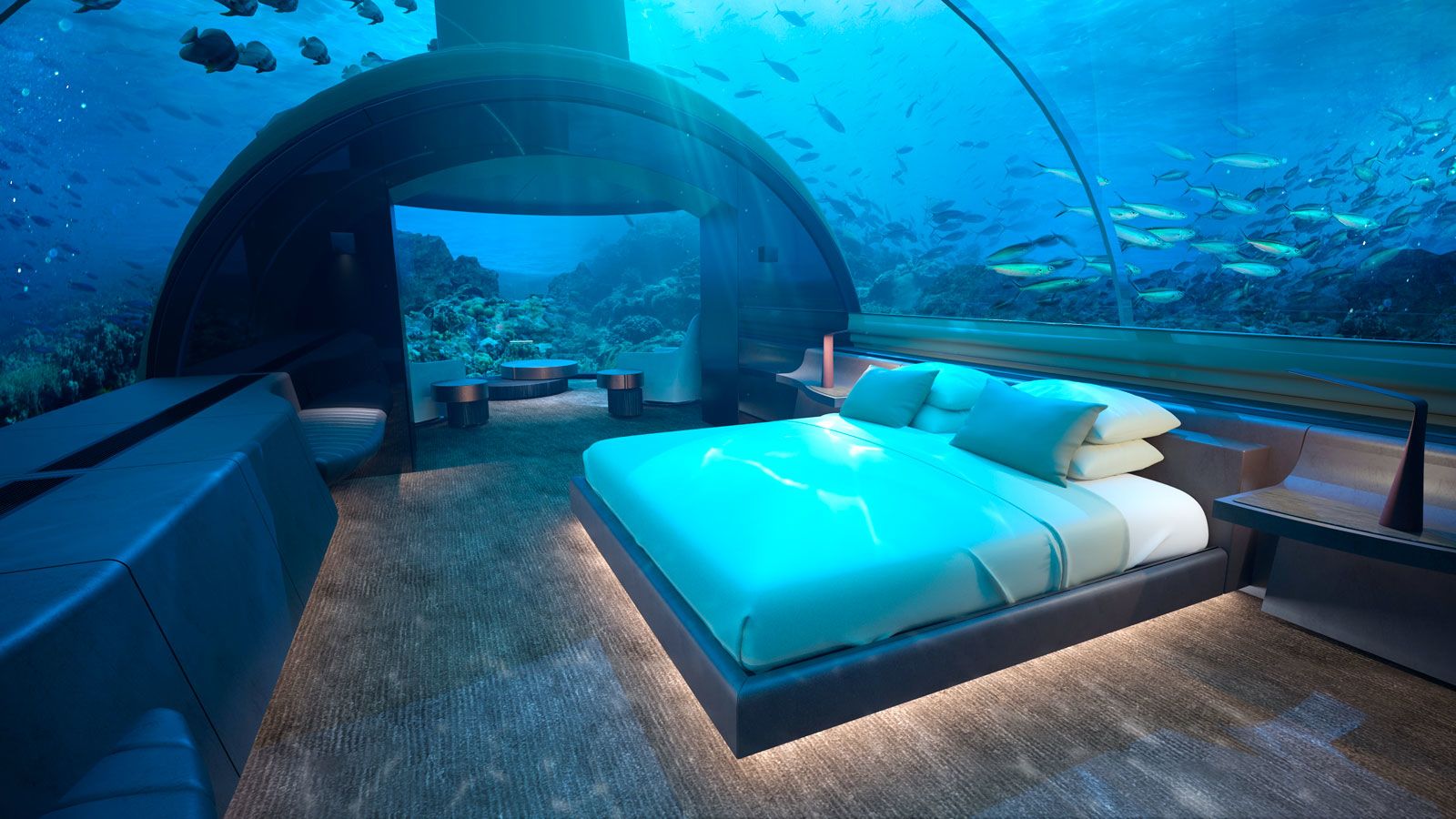The image depicts an enchanting undersea bedroom encapsulated within a glass dome, offering a panoramic view of the seafloor teeming with marine life. Light filters into the room through the dome, casting ethereal shafts of illumination. The centerpiece of the room is a neatly made bed with a black base, crowned by green covers and adorned with six pillows in varying shades of white and blue. To the right of the bed stands a small lamp post. The room gives way to an inviting seating area featuring benches, side tables, and a little round table, forming a cozy nook to observe the schools of fish swimming leisurely outside. The entire setting merges modern comfort with the mesmerizing beauty of the underwater world, providing a unique and immersive experience.